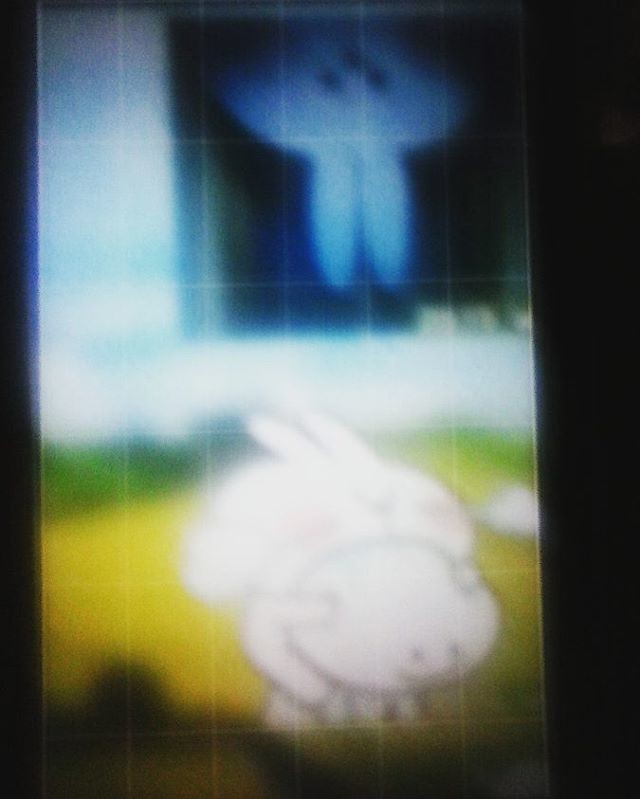In this blurry photograph, a white bunny is depicted prominently, characterized by its long ears and round face. The image is framed by a thick black strip on the right, transitioning to a shaded black on the left, with a hint of blue towards the center. The bunny appears to be positioned at the bottom or middle of the frame, with one of its little arms visible. A yellow hue behind the bunny suggests grass or a similar background element, which is further complemented by green, possibly indicating more foliage. Above this, the sky is represented in various shades of blue and white. The scene includes a dark blue box, within which the bunny appears upside down, with its ears at the bottom. You can also discern the details of the bunny's head, eyes, and nose. The entire image seems to be viewed through a screen or transparent layer, with numerous thin, white horizontal and vertical lines crisscrossing the surface, adding to the overall obscurity.